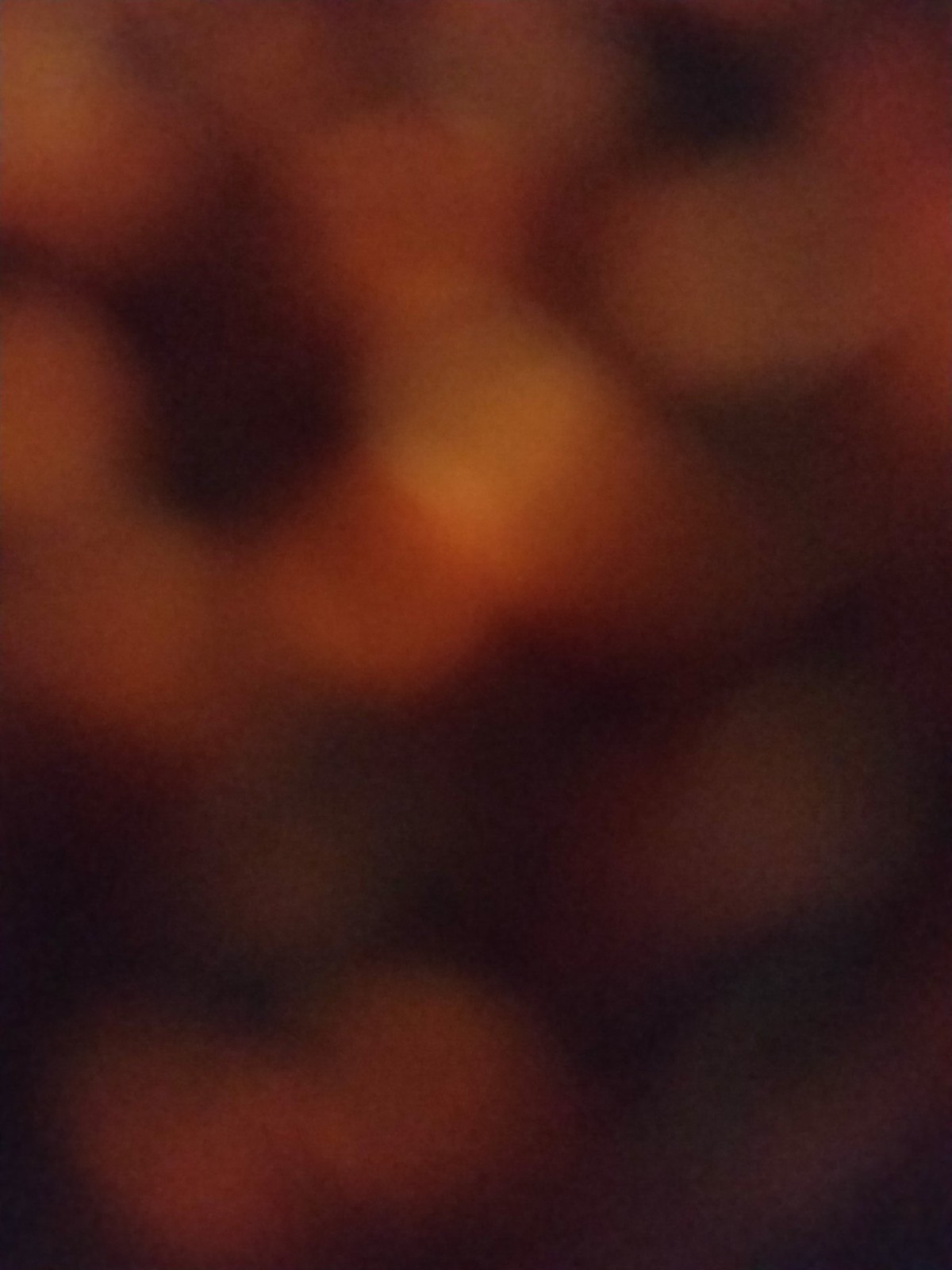This image is a highly blurred and ambiguous close-up, with hints of various objects and colors. The predominant tones are neutral, featuring hints of beige, burgundy, and a significant amount of black in the background. A distinctive white speck occupies the center, serving as a focal point amidst the blur. The scene exudes a natural, almost fleshy palette, reminiscent of a close-up of skin or the front of a hand. Some interpretations suggest the presence of lights, possibly within a dim or varied lighting environment, contributing to the hazy effect. The upper left section features a notable dark spot, likened to a cavity, while the central area presents a raised, flesh-colored segment that could resemble a distorted nose. Despite various guesses, the image remains enigmatic, with elements suggestive of both organic and artificial forms.